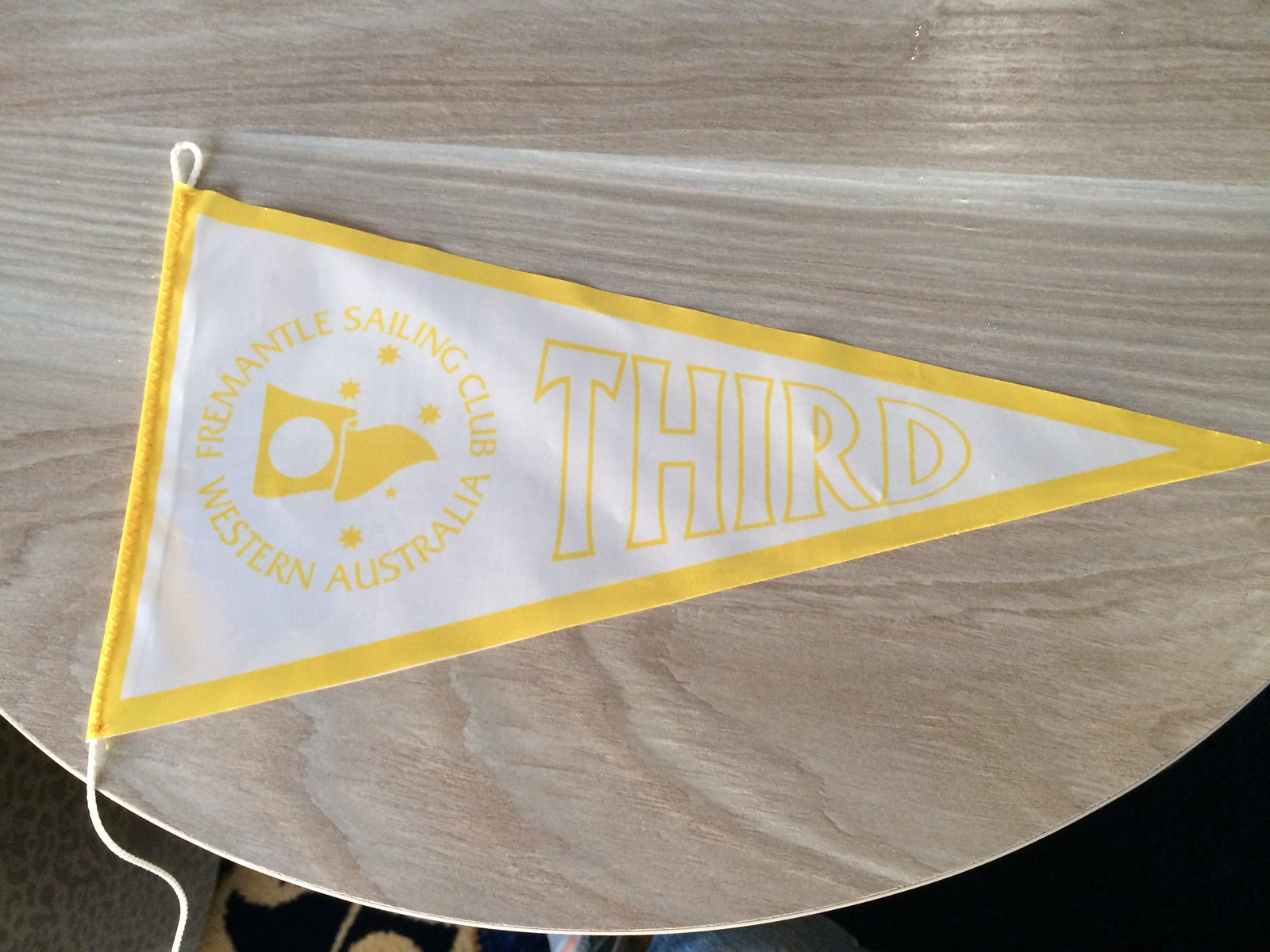The image depicts a group of people under a long shelter, with a wooden table partially visible in the foreground. On the table rests a triangular flag, featuring a prominent yellow border and a white background. The flag is emblazoned with yellow text and symbols. Encircling the central design, the words "Fremantle Sailing Club, Western Australia" are inscribed. At the tip of the triangle, the word "THIRD" is written in capital letters with a hollow, outlined font. The emblem includes a stylized sail and four yellow stars, indicating that this flag serves as a trophy for achieving third place. The detailed patterns on the table suggest it is laminated with a light brown, sandy-colored finish. Although the people in the image are mostly obscured, a hint of a body, presumed to be a woman, is visible, hinting at minimal human presence.